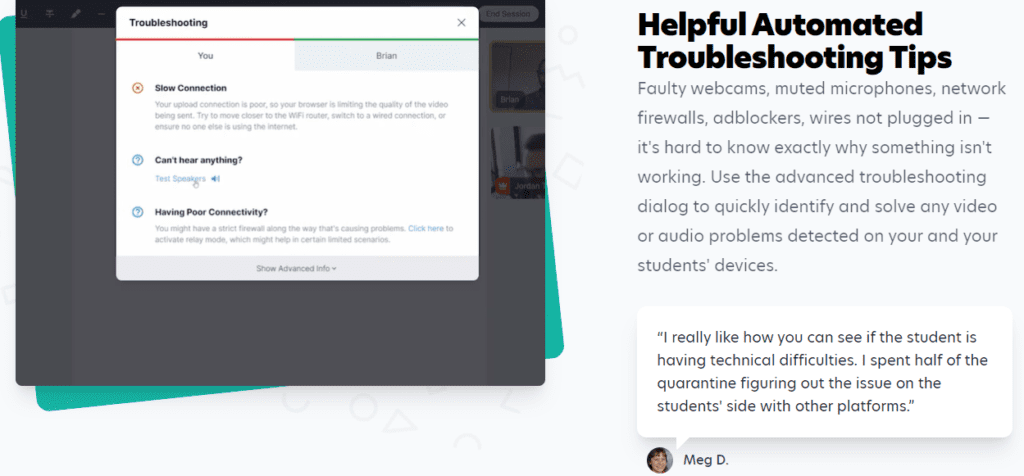This image, captured from a computer screen, features a complex layout prominently showcasing a troubleshooting interface. In the background, there is an off-centered, tilted teal square with its corners and edges visible, except for the upper right corner where the teal is excluded. Overlapping the teal area on the left, there is a larger gray screen, which is then covered by a white rectangle labeled "Troubleshooting."

Inside the white rectangle, at the top, "You" is written in red, next to "Brian" in green. Below these names, there are three possible issues listed: "Slow connection," "Can't hear anything," and "Poor connectivity."

To the right of this main section are a couple of paragraphs providing additional explanations. This section is topped with the bold black header "Helpful Automated Troubleshooting Tips." At the bottom, a user testimonial by a woman named Meg D. is included. She states, "I really like how you can see if the student is having technical difficulties. I spent half of the quarantine figuring out the issue on a student's side with other platforms."